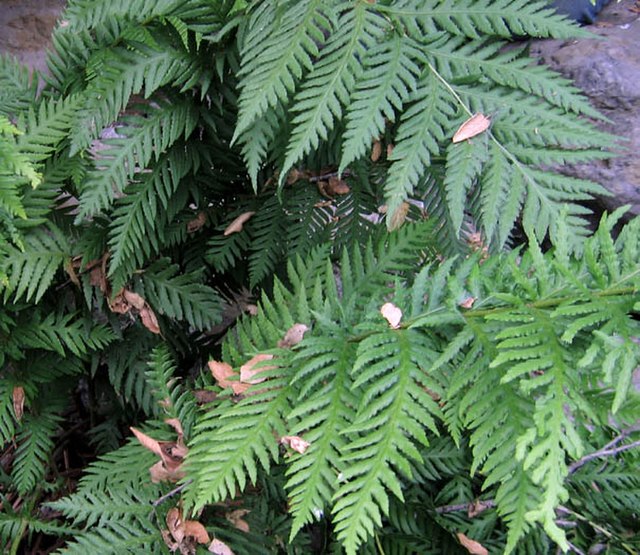This photograph captures a close-up of vibrant green fern leaves, each characterized by a central stem from which smaller, serrated sections branch out, giving the appearance of long tapered leaves. The ferns are densely clustered, creating a lush foreground, interspersed with smaller, dead brown leaves that have fallen from another plant. These smaller leaves contrast sharply with the green, adding texture and detail to the image. In the background, dark brown rocks, tinged with a hint of pink, define the top left and right corners, indicating a natural, outdoor setting. Subtle hints of stone and ground are visible beneath the ferns, and a blue material, possibly someone's pant leg, peeks in at the top right, suggesting human presence. The photograph is taken during the daytime, capturing the intricate details of the fern leaves against the rocky backdrop.